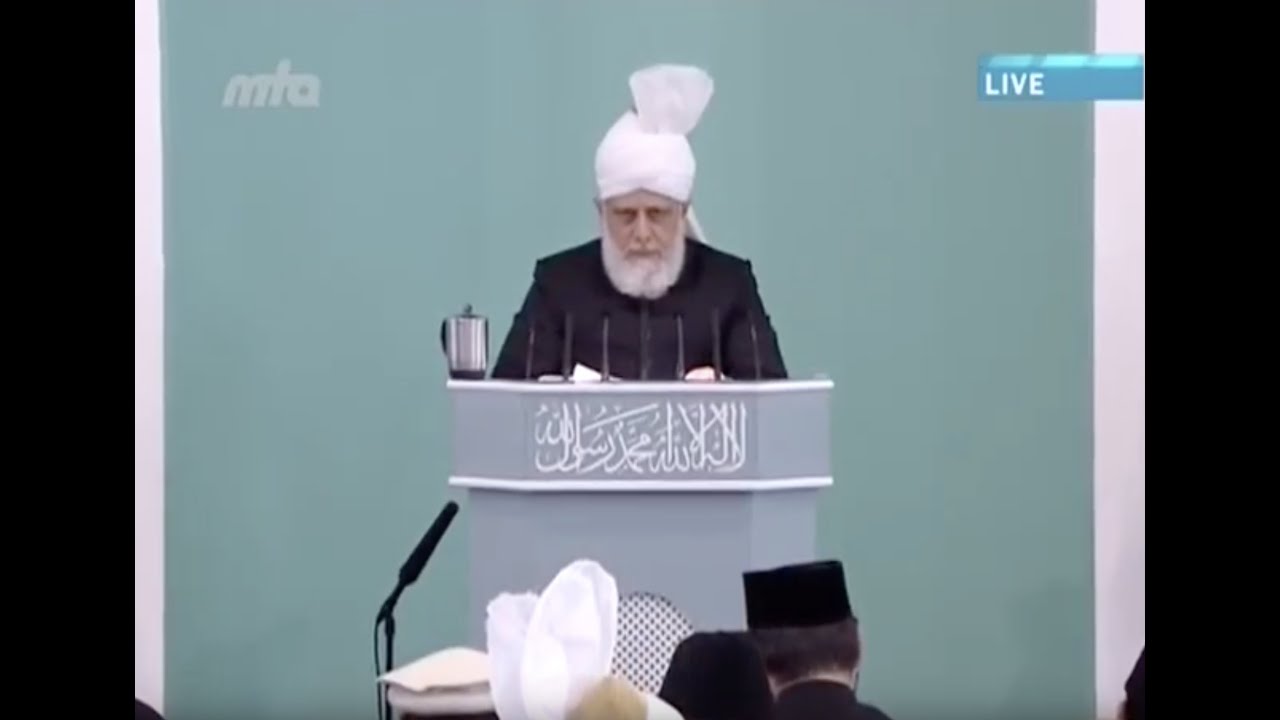The image captures a low-quality screen capture of a television broadcast. At the heart of the image, a middle-aged Middle Eastern man stands behind a light gray podium embellished with white stripes at the top and bottom. The podium is adorned with white text in what looks like Arabic script. The man, centered in the image, dons a white headdress and has a prominent white beard. His attire includes a long-sleeved dark shirt, seen from the chest up.

In front of him on the podium, there is an assortment of thin microphones with black tips and a small pot positioned to the left. He appears to be giving a press release or news report, illuminated by a greenish-aqua screen set behind him, which is bordered by white strips that end in black bars on the sides of the image.

The top corners of the image feature text: the upper left corner displays a watermark reading "MTA," while the upper right corner has a TV graphic with the word "Live" in white. The bottom of the image reveals the back of several listeners' heads, including a person with short brown hair and a black rectangular hat to the right of the podium, along with what seems to be another individual with a white hat slightly off the edge of the frame. A boom mic also angles towards the speaker from the left side of the image.